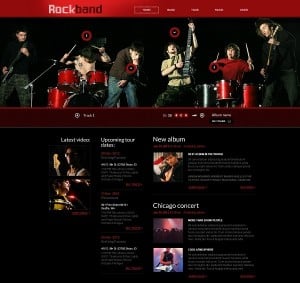The website features an eye-catching design with a dark red, shiny banner at the top that prominently displays the name "Rock Band." The word "Rock" is in a lighter color compared to "Band." This banner also includes a navigation bar with five options, including "Home" and other essential pages for easy access.

The top portion of the website showcases an image of a vibrant band performance. In the background, two drummers, each playing red drums, can be seen. A guitarist, dressed in a black shirt and camo pants, stands to one side. At the forefront, a vocalist wearing blue jeans and a gray shirt takes center stage with a microphone, while a drummer in a red shirt energetically plays in the back.

The bottom section of the website is dominated by a sleek, black background, featuring a "Latest Videos" section listing various new video content. Adjacent to this section, there's a highlight of a new album, complete with an image of the album cover and some accompanying text information to the right. Beneath this, there's a mention of a "Chicago Concert," with two related photographs. The first photo captures a lively concert crowd, and the second shows a musician holding a white electric guitar, each with descriptive text beside them.